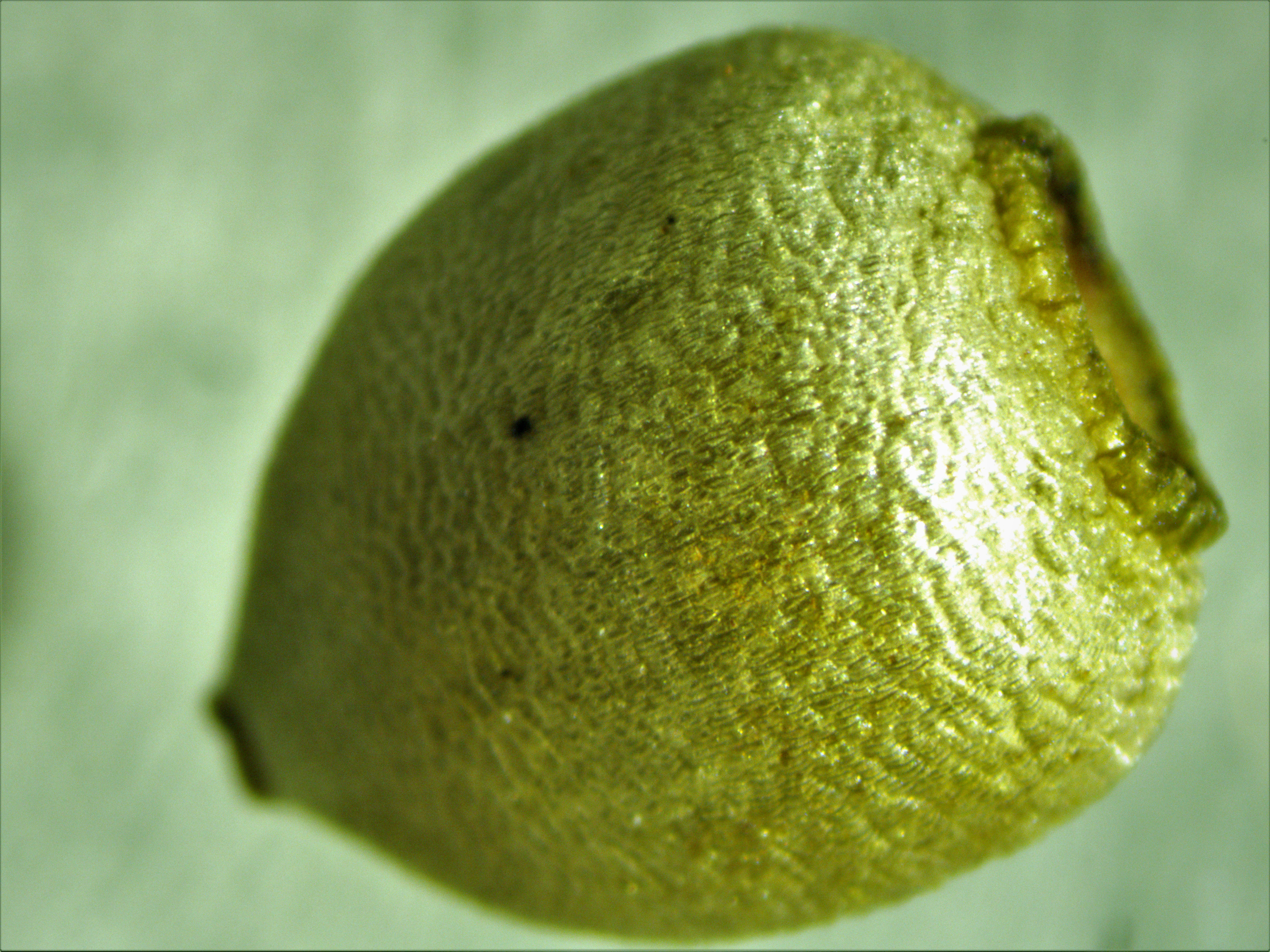This image presents a highly detailed close-up of a fruit-like or pod-like green structure, positioned centrally against a blurred, somewhat transparent green background. The object resembles a lime in its bumpy texture and shape but might not be one. It features an open hole on the right side, exposing a vaguely hollow interior. Light hits this object from the right, resulting in a gleaming shine. Noteworthy is the presence of small black or dark brown spots, possibly indicative of mold or imperfections on its surface, particularly a notable dark spot slightly to the left of center. The top end of the structure appears to have a smaller opening where it might have been attached to a stem, or it could be the point from which seeds were dispersed, suggesting it could be a seed pod. The overall visual emphasizes the central object with no additional elements in the frame, focusing on the intricate details, textures, and irregularities of this mysterious botanical specimen.